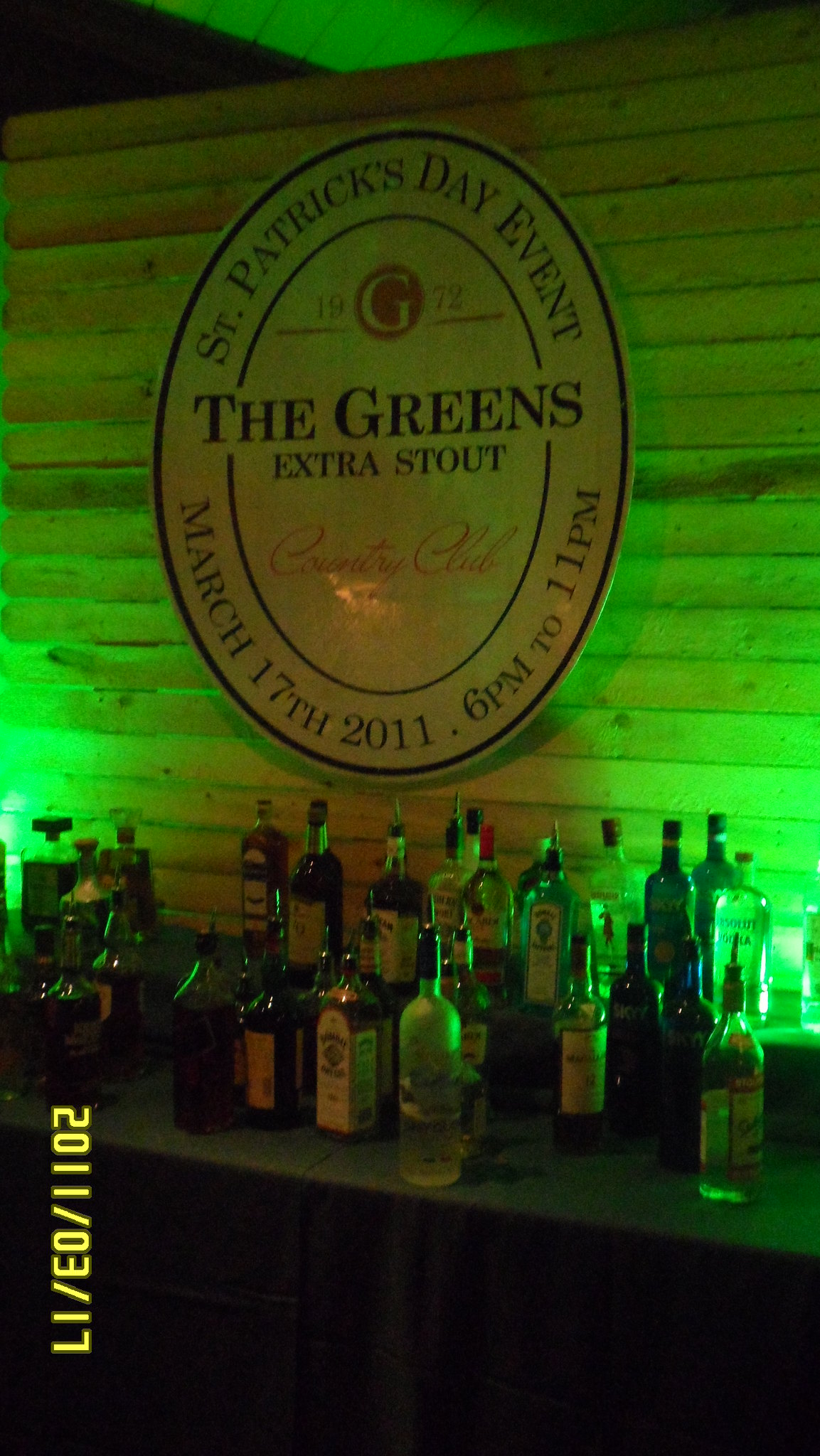The image depicts a St. Patrick's Day event at a bar, highlighted by a prominent, backlit wooden wall illuminated in vibrant green lights. The centerpiece of the wall features a large, white logo with bold black letters that read "St. Patrick's Day Event" and "1972, The Greens Extra Stout." Beneath this, in cursive script, it says "Country Club," though the words are partially obscured. The event details—March 17, 2011, from 6 p.m. to 11 p.m.—are clearly marked. In front of the wall, a multi-leveled bar countertop is crowded with an impressive array of liquor bottles, including popular brands like Grey Goose, Bombay Gin, Beefeater, and Absolut. The entire scene is bathed in green light, enhancing the festive atmosphere. A digital timestamp, "2011-03-17," is visible on the side of the photograph, most likely added by the camera.